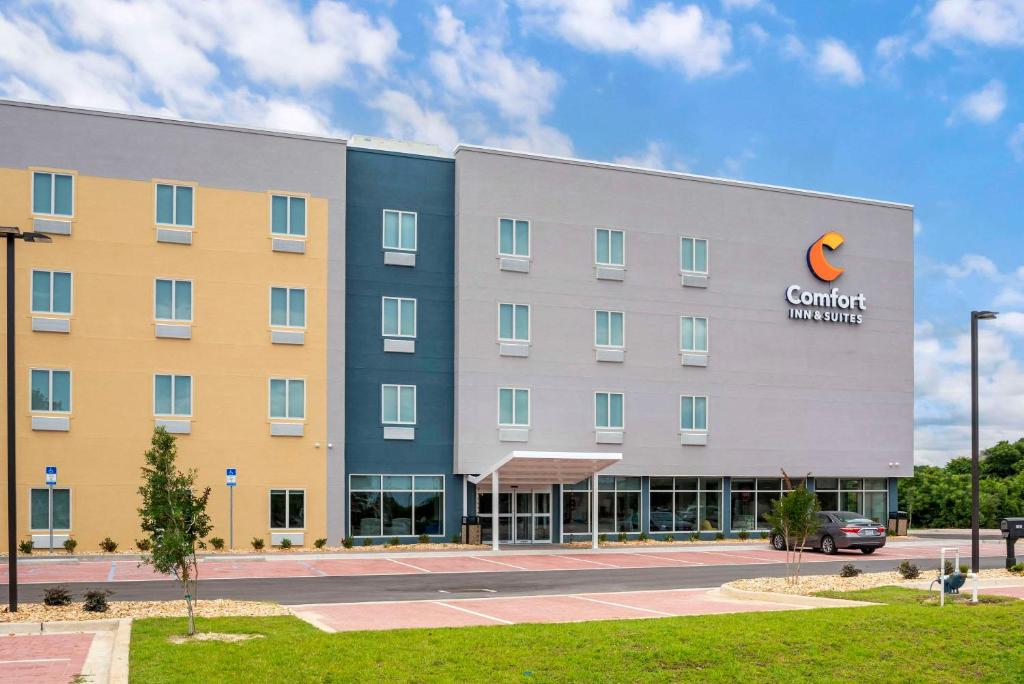The image depicts the Comfort Inn & Suites hotel, captured from an angled, front-facing view. Dominating the middle background, the hotel is a lengthy rectangular structure. The right portion of the building displays the recognizable orange and yellow "C" logo in the upper right corner, with "Comfort" in large white font and "Inn & Suites" beneath in smaller text. This section of the building is predominantly gray, transitioning to a tall, thin bluish area to its left, with three vertically aligned windows framed in white. The leftmost part of the building is primarily yellow with a gray border on the top and sides. 

All windows on the hotel are tall, rectangular glass panes, consistently featuring white trims. In the front, there's an additional row of windows and a large white awning over automatic sliding doors, welcoming guests. Below the clear blue sky, the foreground includes a neatly spaced parking lot with spaces marked in salmon color and white lines. A single car is parked in the bottom right, beside a light pole, all accentuated by patches of lush green grass surrounding the parking area. The entire scene is bathed in daylight, highlighting the hotel's facade and surroundings vividly.